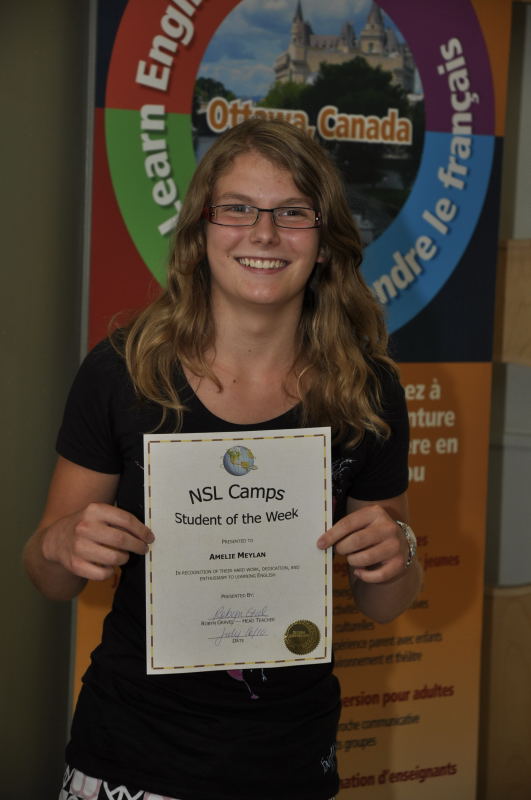In this indoor photo, a young woman with wavy, light brown hair that falls just below her shoulders is standing and smiling broadly. She is wearing a black short-sleeve shirt and rectangular black-framed glasses. In her hands, she holds up a certificate that reads, "NSL Camps Student of the Week, presented to Amelie Malin." The certificate appears to feature a handwritten signature and a date. She is also wearing a silver watch on her left wrist. 

Behind her is a large, multicolored sign featuring a circular design divided into four quadrants: red in the upper left, purple in the upper right, blue in the lower right, and green in the lower left. The sign has partially visible text, with "Learn English" written in white and additional text in French. At the center of the sign is an image of a large building, and above it, in orange lettering, are the words "Ottawa, Canada." The background suggests that this photo might be taken in a Canadian educational setting where multiple languages, particularly English and French, are promoted.